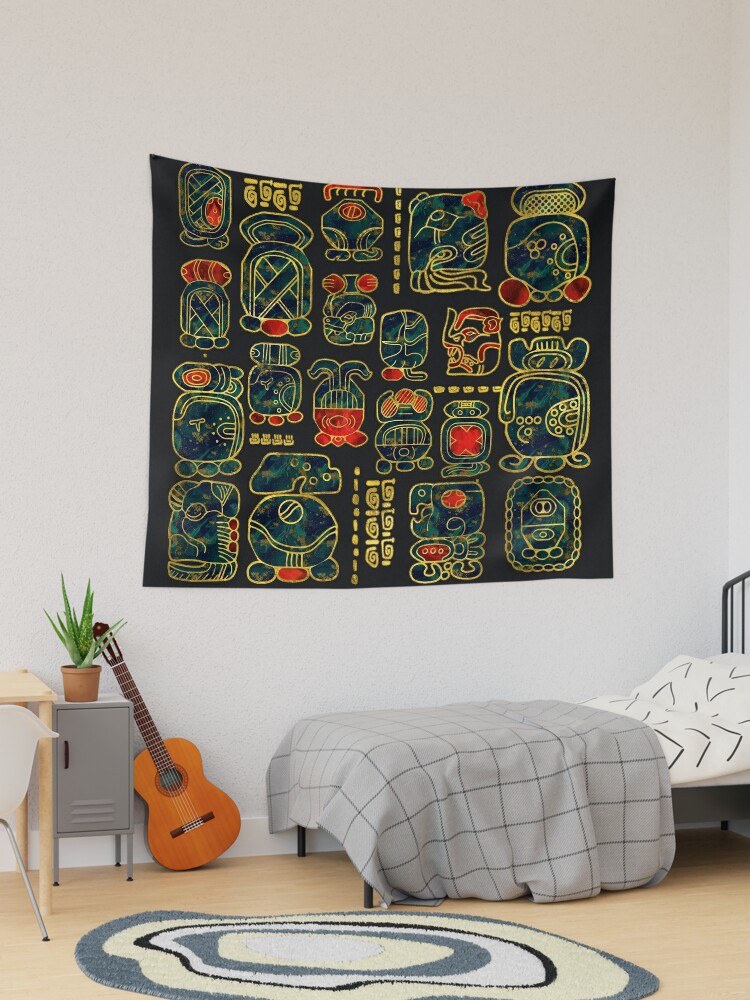The image depicts a detailed mock-up of a bedroom, likely belonging to a teenager or child. The room features a twin bed with a black iron frame pushed up against a gray wall. The bed is adorned with white sheets that have black arrows and black bee designs, and a gray and black plaid blanket is draped over it. Adjacent to the bed is a small, gray nightstand designed to look like a high-school locker, with a terracotta pot containing an aloe vera plant on top. Leaning against the nightstand is a small, very orange acoustic guitar.

The floor is made of natural wood tiles, and an oval-shaped rug with concentric, misshapen ovals in shades of blue, cream, black, and white lies comfortably in front of the bed. There is also mention of a circular rug, indicating the possibility of multiple floor coverings.

A natural wood desk with a white plastic chair featuring metal legs is also present in the space. On the wall hangs a striking black tapestry with various tribal symbols in blue, red, and yellow. The description brings attention to repeated elements such as the orange guitar and the black blanket with numerous designs, emphasizing their prominence in the room’s overall aesthetic.